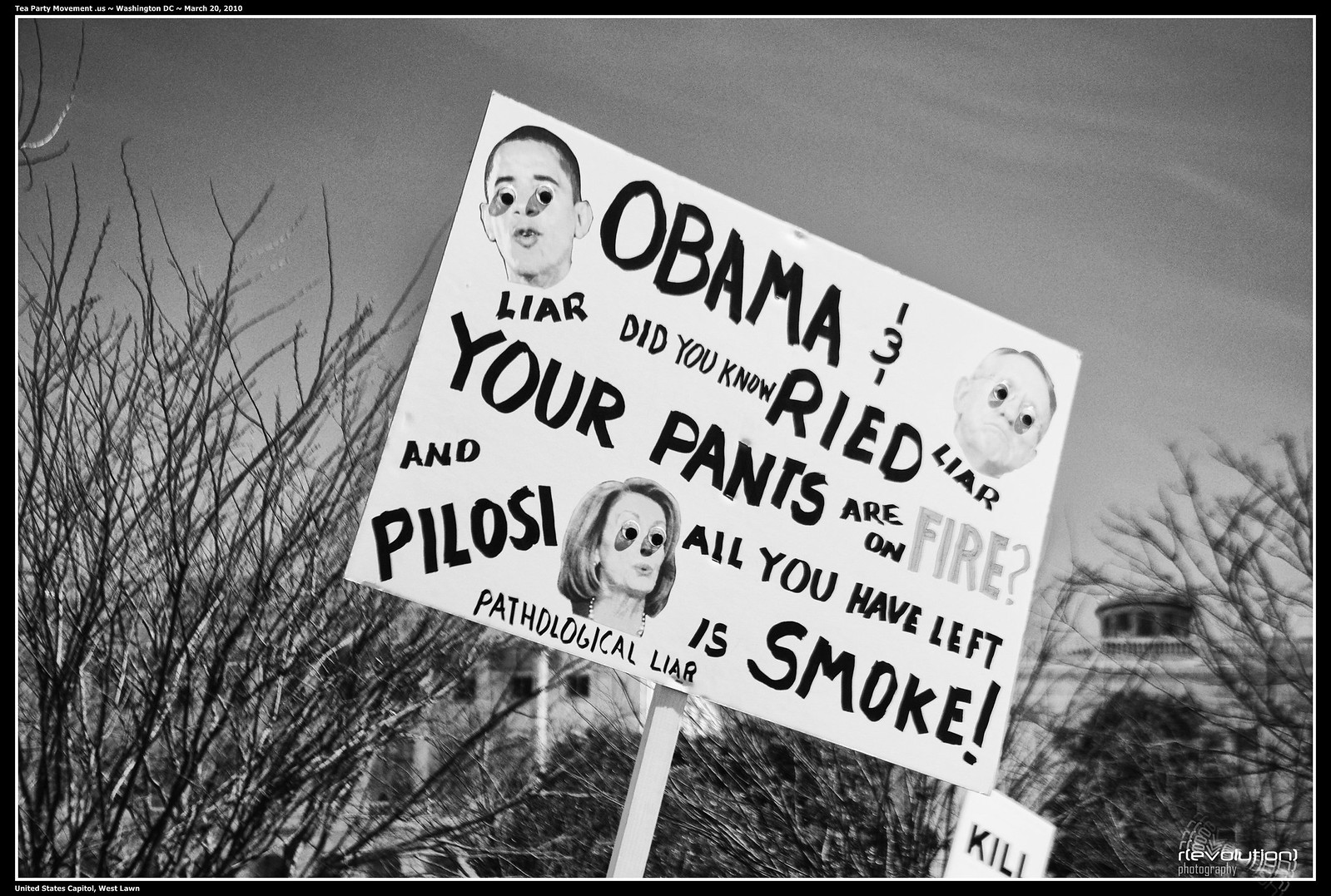This horizontally aligned rectangular black-and-white image is bordered by a thick black edge with a thin white inner outline. The sky in the background appears gray with swirling clouds. In the foreground, leafless bushes are silhouetted against the sky. The focal point of the image is a handwritten protest sign mounted on a wooden plank. The sign is prominent in the foreground, featuring a blend of text and drawn faces with exaggerated "googly eyes" of prominent figures including Obama, Nancy Pelosi, and another male figure, possibly Senate Majority Leader Harry Reid (mistakenly referred to as "Reed"). The sign reads, "Obama and did you know your pants are on fire?" followed by, "Pelosi, all you have left is smoke." Below Obama's image, it says "LIAR," and beneath Pelosi's headshot, it reads "pathological liar." The backdrop features the White House, slightly obscured by leafless trees. At the very top left corner, tiny white text states, "Tea Party Movement, Washington D.C., March 20, 2010," and in the bottom left corner, it reads “United States Capitol, West Lawn.” The words on the sign appear to be handwritten, and there's a minor, partially legible sign in the lower right, potentially reading "KIL."